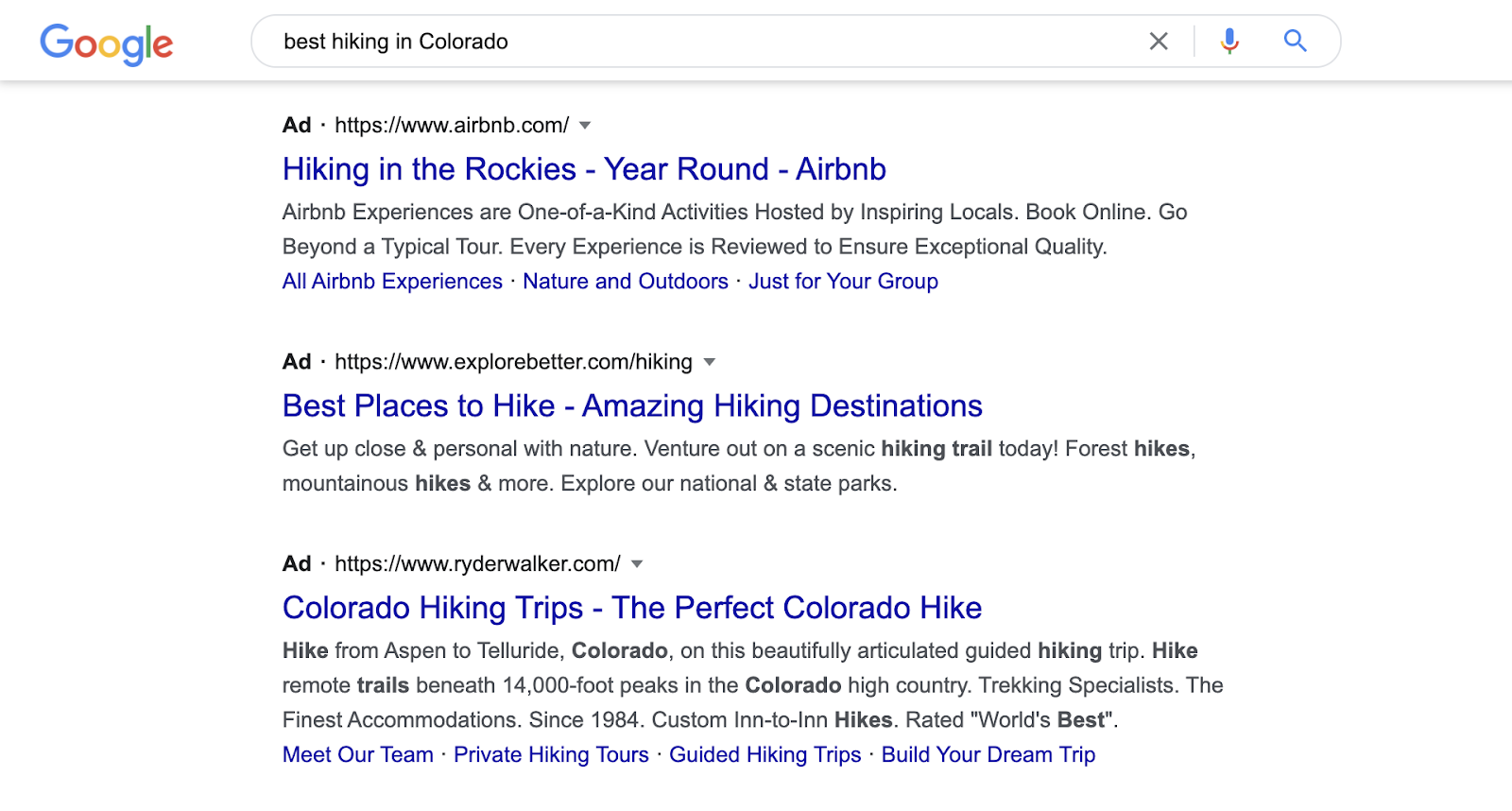This image is a screenshot of a Google search results page on someone's computer, displaying the query "best hiking in Colorado" in the search bar at the top. The Google logo, featuring its distinctive rainbow colors, is visible in the upper left corner. Below the search bar, the top result is an ad from Airbnb, which includes the URL airbnb.com and the headline "Hiking in Rockies Year-Round Airbnb," followed by a brief description in black text.

The second result is another ad, this time from explorebetter.com, with the blue headline "Best Places to Hike Amazing Hiking Destinations," accompanied by additional text in black. The third result is an ad from riderwalker.com, featuring the blue headline "Colorado Hiking Trips The Perfect Colorado Hike," and further descriptive text underneath.

Additional clickable blue text on this result includes options such as "Meet Our Team," "Private Hiking Tours," "Guided Hiking Trips," and "Build Your Dream Trip." The screenshot reveals that the initial Google search for the best hiking in Colorado has predominantly returned ads for various websites offering hiking trips and related services.